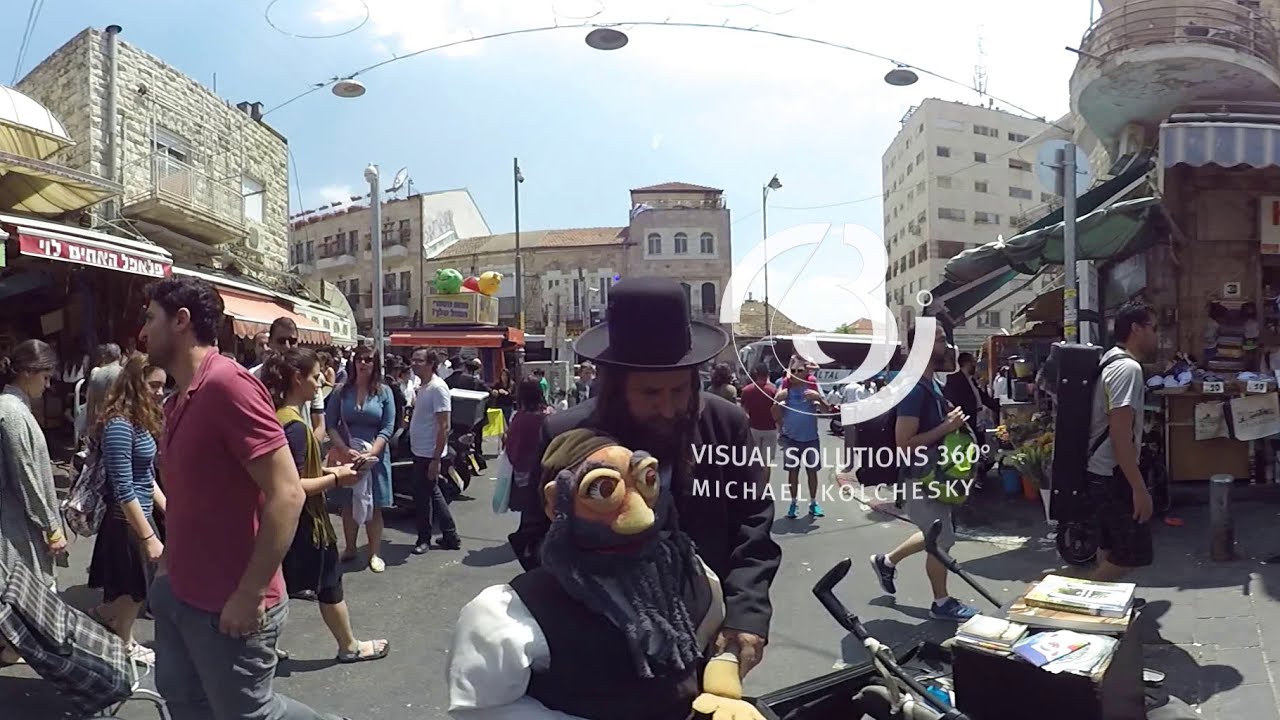The image depicts a bustling outdoor marketplace in a foreign country with numerous small shops and people walking up and down the street. Prominently in the center, there's an Amish-looking man wearing a black hat and coat, holding a large puppet with exaggerated features – a large nose, big eyes, and a black beard. To his left, a man in a maroon T-shirt and a woman in a blue shirt and black skirt can be seen. There's a noticeable variety of buildings; smaller shops line the street, while larger, older gray buildings, possibly apartment complexes, stand in the background. Overhead, a string of circular lights runs through the market area. Among the lively crowd, two men on the right side carry heavy backpacks and wear shorts. The blue sky with a few clouds illuminates the scene, and there is a watermark on the image that reads, "Visual Solutions, 360 degrees, Michael Kolchesky."